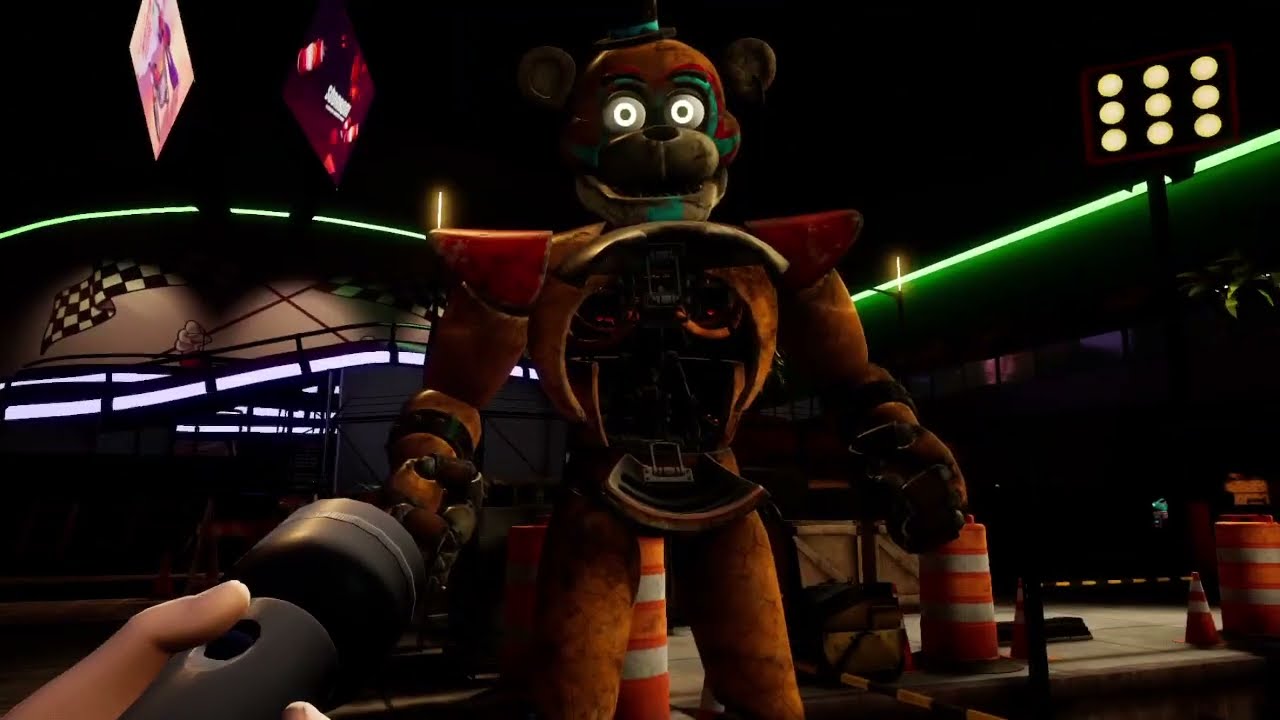The image is a dark, animated scene resembling either a video game or a computer-generated movie, likely inspired by the Five Nights at Freddy's franchise. Dominated by black tones, the wide, horizontal frame is punctuated by selective lighting. Neon signs in the top left and a stadium light setup with nine golden circles at the top right contribute to the eerie ambiance. The background is further illuminated by swirling neon lights and striped orange-and-white road cones, evoking a construction zone setting.

Front and center stands a bear-like animatronic character with human characteristics. The creature is covered in red-brown fur, with eyes glowing golden yellow outlined in green, exuding a sinister, almost possessed demeanor. A small black top hat with a green band sits atop its head. The bear's arms are extended forward, and its mouth is open, revealing sharp details. Notably, its chest has a circular opening, suggesting it has been gutted or requires an insertion.

In the bottom left corner of the image, an animated human hand holds a black flashlight, directing its beam towards the bear animatronic, highlighting its ominous presence in the dark, shadowy room.